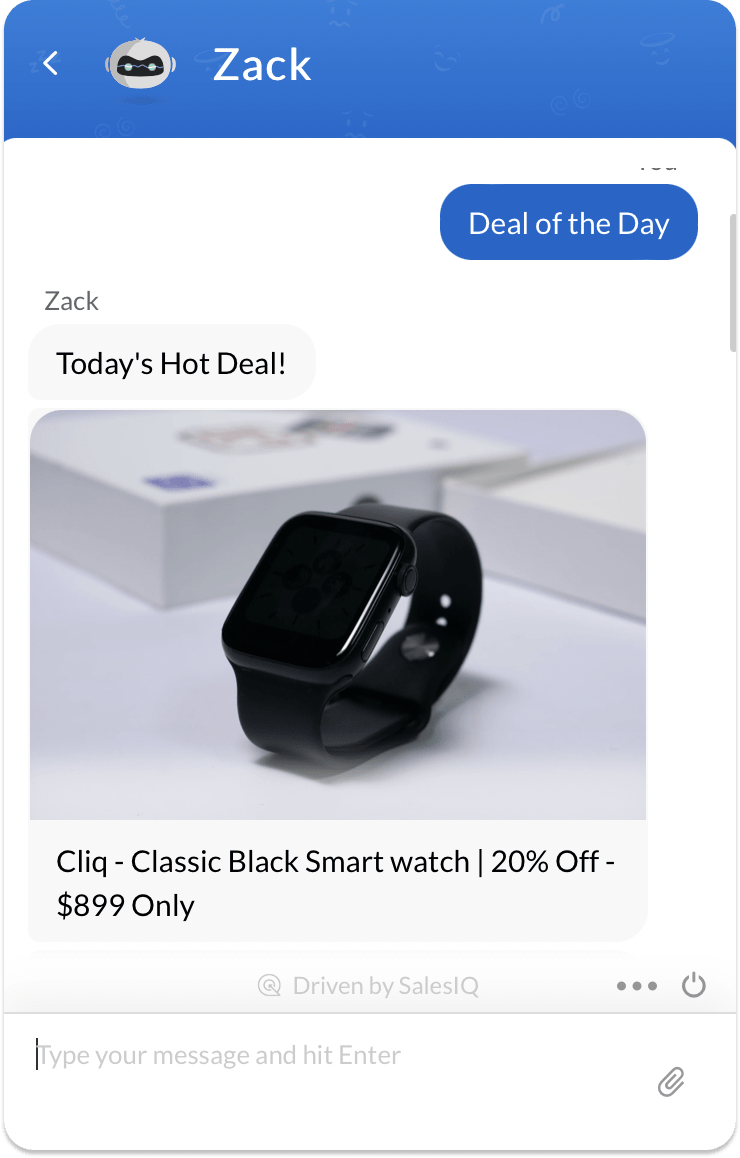This is a detailed screenshot showcasing a promotional offer for a smartwatch. The screenshot appears to be from a messaging app, where a user named Zach has shared today's hot deal. The central focus of the image is a sleek, black smartwatch with a matching black band. In the background of the image, the smartwatch's white packaging box is partially visible, enhancing the presentation of the product.

Beneath the image, there is a succinct description stating "Classic Black Smartwatch 20% off - $899 only," highlighting the discounted price. The messaging app interface includes a prompt at the bottom, ready for the recipient to type a reply. Prior to Zach's message, the text "Deal of the Day" is visible, suggesting that this message thread features daily deals that users can interact with to receive special offers. The overall scene effectively conveys the excitement of an exclusive discount in a user-friendly communication format.